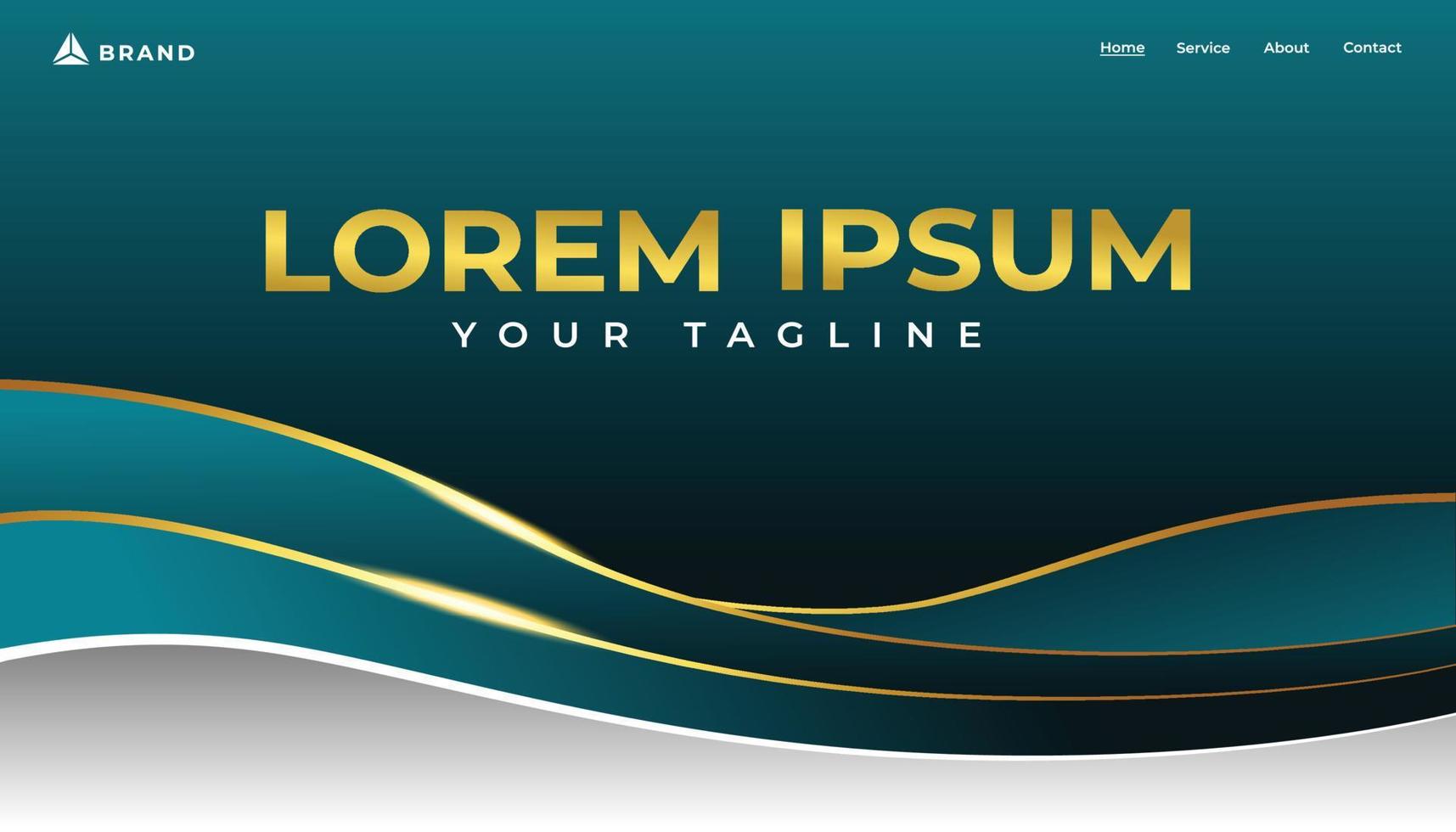This image showcases a proposed design for a web page template, primarily intended as a homepage for a business website. The layout features a distinct, visually appealing wavy design characterized by various shades of green, transitioning from a dark green at the top to lighter, blue-green and pale green hues towards the bottom. Gold lines, including wavy ones, accentuate the sections and add an elegant touch, while a single wavy white line and a gray panel demarcate different areas of the page.

At the very top of the page, a triangular pyramid logo sits next to a placeholder text labeled "brand" in white, indicating where a company’s logo would be displayed. To the upper-right corner, a navigation menu bar provides links to "Home," "Service," "About," and "Contact" pages, offering easy access to essential sections of the site.

Dominating approximately two-thirds of the central area against the dark green backdrop is large, gold placeholder text stating "Lorem Ipsum." Beneath it, in smaller white letters, reads "Your Tagline," serving as placeholders for the company name and tagline, respectively. This highly detailed and stylized template effectively demonstrates how one might customize and fill in the content to create a personalized and professional web page.